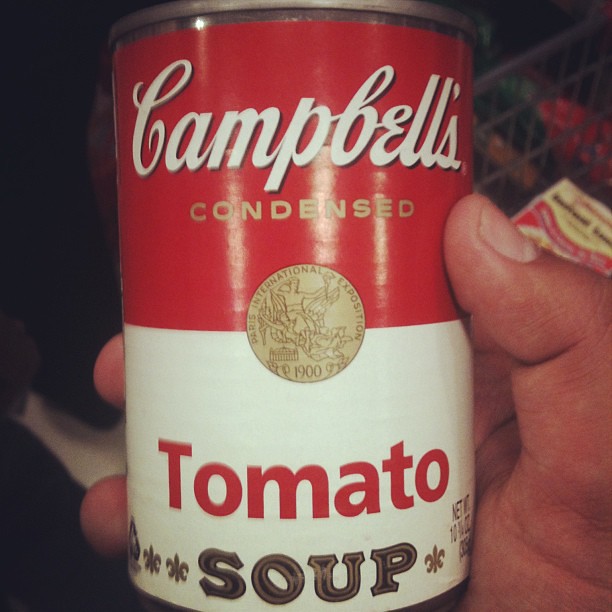The image depicts a close-up of a person's right hand, appearing to be a man's hand, holding a can of Campbell's condensed tomato soup. The upper half of the can's label is red, and the lower half is white. Prominently, the word "Campbell's" is written in white letters on the red background. Below it, "condensed" is inscribed in gold. "Tomato" is displayed in red text on the white portion of the label, while "soup" is in black with gold trimming. In the center of the label, there's a small circular gold badge featuring an image from the Paris International Exposition 1900, showing a figure, possibly Caesarean, on a platform or bed carried by servants. At the bottom corners near the word "soup," there are small symbols resembling flowers. The background of the image hints at the presence of a box of instant ramen noodles in a Styrofoam container.